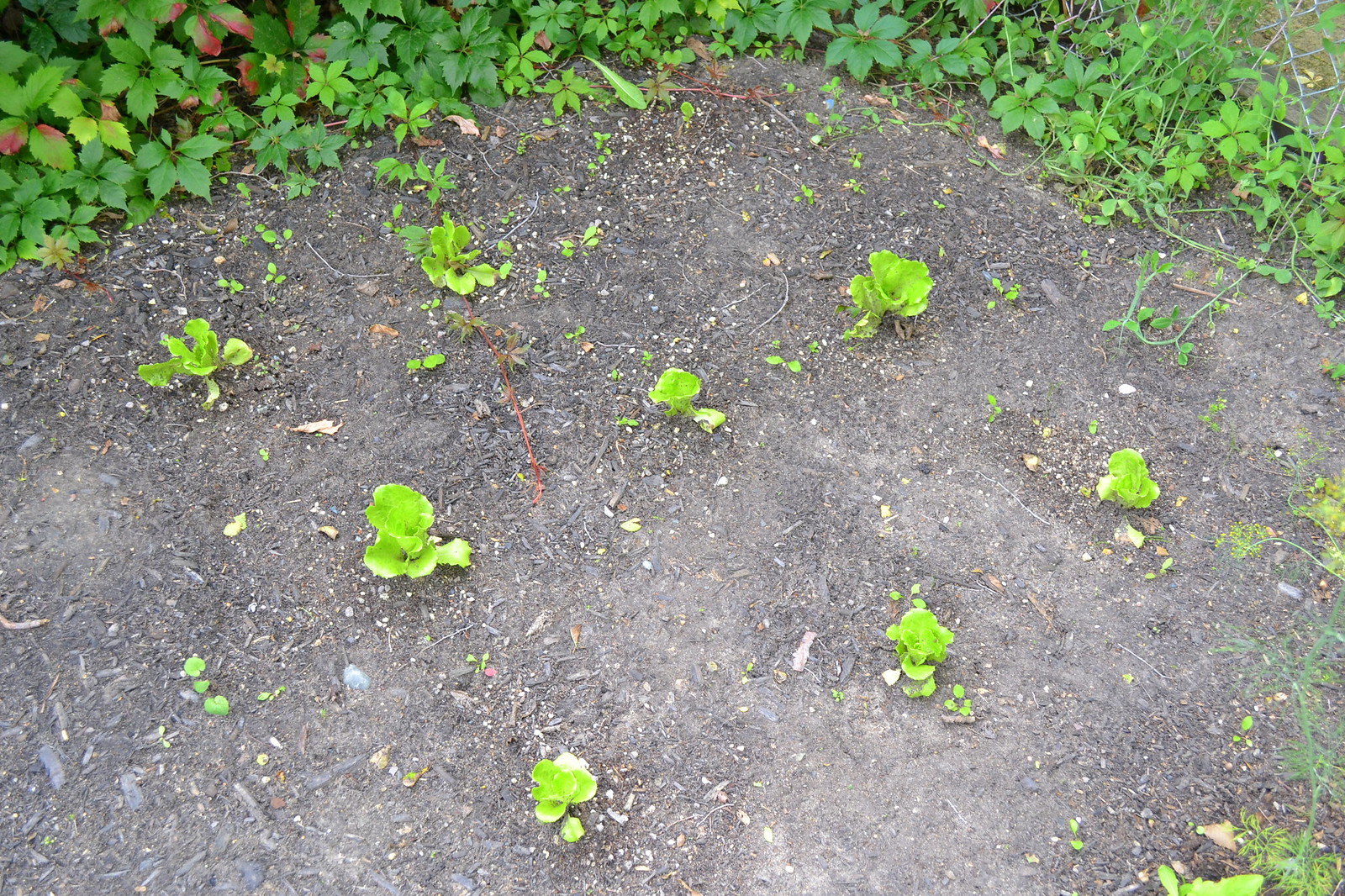This photograph captures a top-down view of a vegetable garden immersed in rich, brown soil. The central focus is a patch of mostly bare, cultivated earth, punctuated by orderly rows of young, leafy green plants that are likely cabbage or lettuce, planted for food purposes. Each plant boasts star-shaped, light green leaves, indicating they are still in the early stages of growth. Surrounding this cultivated patch, a variety of vines and ground cover vegetation create a natural boundary. The garden's perimeter is defined by a chicken wire fence, at the base of which these additional plants thrive. The soil appears rich and well-tended, perhaps previously mulched. The photo, taken on a clear sunny day, showcases a tranquil outdoor scene dedicated to cultivation amidst nature.